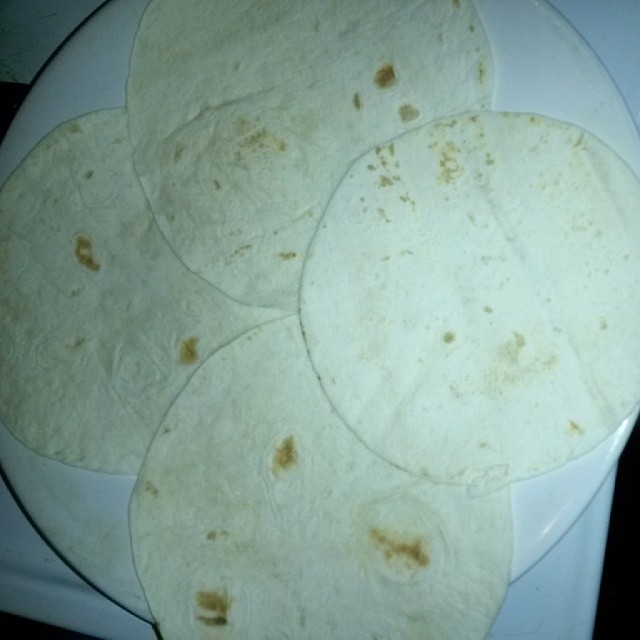This overhead image showcases a white ceramic plate adorned with four flour tortillas against a backdrop that includes a slightly visible black underlay and either a white tablecloth or placemat. The tortillas, featuring an off-white hue with scattered brown spots indicative of cooking, overlap at the center, creating a formation reminiscent of a four-leaf clover or a plus sign. Each tortilla displays varying degrees of browning and minor wrinkles, emphasizing their texture. Notably, the arrangement sees the right-side tortilla positioned above the rest, with the top and bottom tortillas layered beneath it, and the left-side tortilla at the very base. The platter itself has a distinctive round shape towards the top, transitioning into a more square-like form near the bottom, with the top-right edge worn or discolored, adding subtle character to the image.